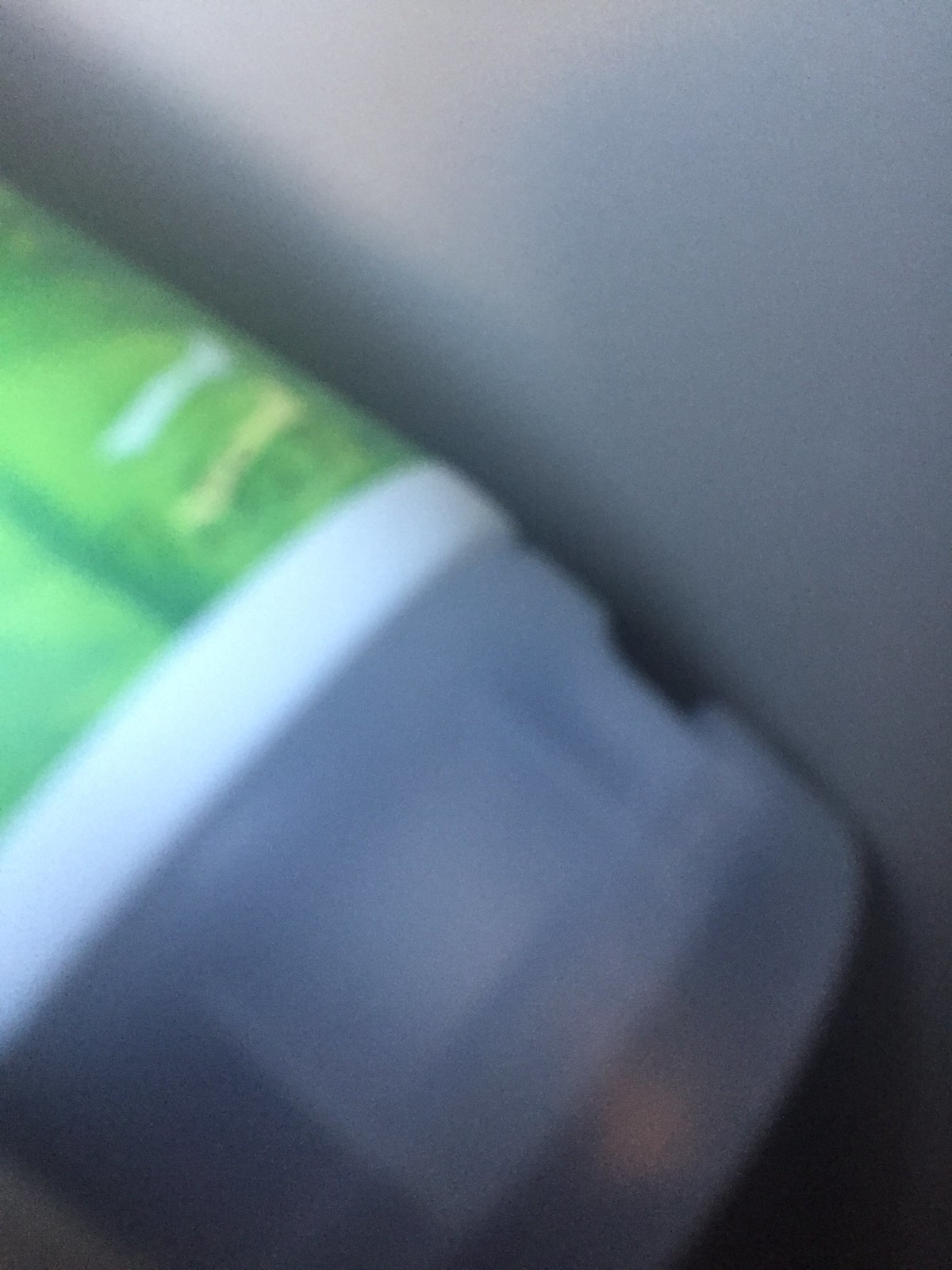A close-up, slightly blurry image captures a green cylindrical bottle at a slant, extending from the upper left corner towards the lower right corner of the frame. Just before the lower right corner, there is a shadow cast by the bottle, creating a dark patch. The upper right section of the image includes the edge of a white table surface, which the bottle is resting on. The green bottle features a white rim separating the base from a transparent flip cap.